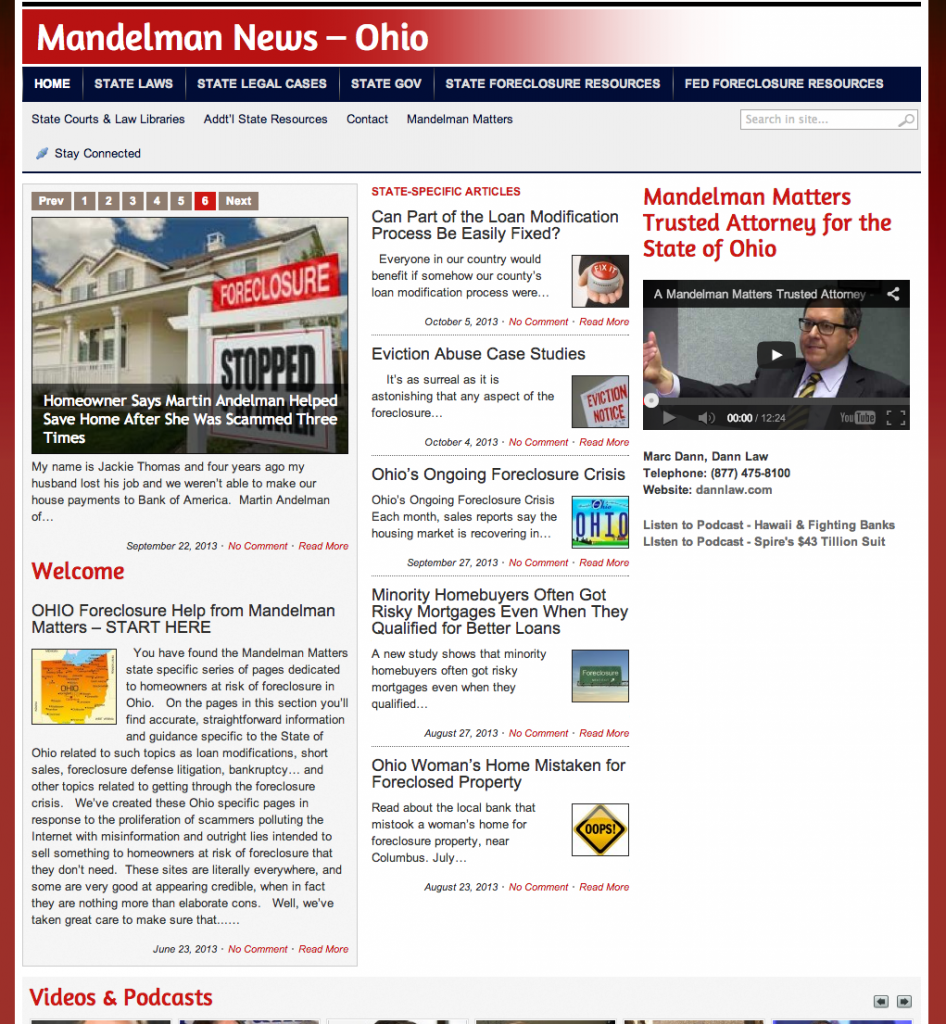A detailed descriptive caption for the image based on the provided voice note can be:

---

The image is a complex screenshot from the news website "Mandelman News Ohio." At the top, a red banner with white text displays the website's name, followed by a very dark blue or black navigation bar with white text listing various sections: "Home," "State Laws," "State Legal Cases," "State Gov," "State Foreclosure Resources," "Fed Foreclosure Resources." Below this, a grey band with black text contains links to "State Courts and Law Libraries," "Additional State Resources," "Contact," "Mandelman Matters," "State Connected," and includes a search bar. 

Prominently displayed on the left side is a series of six pictures, with the sixth image selected. This particular image shows a house with a "Foreclosure" sign marked "Stopped." Underneath, a banner headline reads, "Homeowner Sains Martin Mandelman helped save home after she was scammed three times." Below the banner, there's a section titled "Welcome," next to an "Ohio Foreclosure" help guide with a map of Ohio and extensive accompanying text. At the bottom of this column, partially visible, are tabs for "Videos and Podcasts.”

Central to the screenshot are state-specific articles with highlighted topics: "Can part of the loan modification process be easily fixed?" featuring an image of a person’s hand holding a red and grey round object; "Eviction Abuse Case Studies" illustrated with a red eviction notice; "Ohio's Ongoing Foreclosure Crisis" accompanied by an Ohio state symbol in blue and yellow; and "Minority homeowners often got risky mortgages even when they qualified for better loans," with a green sign on a blue background.

On the right side of the image, a video preview shows a man in a suit and glasses. Above the video, the caption "Mandelman Matters Trusted Attorney for the State of Ohio" is written in red text.

---